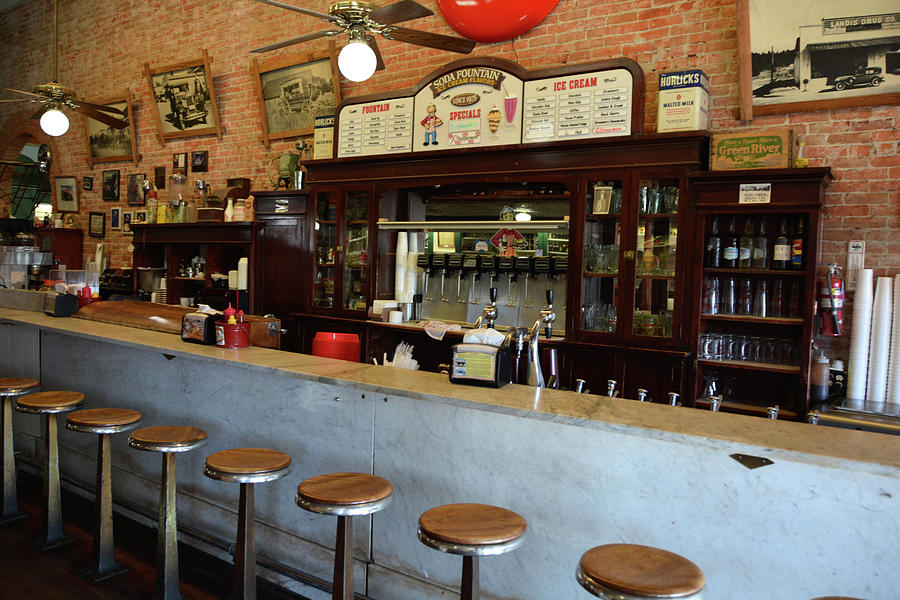This photo captures the nostalgic ambiance of a vintage ice cream parlor and soda fountain, reminiscent of establishments from the early 20th century. The setting features a white counter with a worn wooden countertop, lined with nine barstools. Above the counter, a large sign against a brick wall reads "Fountain" and "Ice Cream" in red letters, flanking a cartoon character with a mustache holding various confections. The high ceiling, adorned with large five-blade ceiling fans and round light fixtures, complements the overall classic aesthetic. The counter holds condiments such as napkins and various flavoring bottles, hinting at the wide variety of sodas and ice cream parfaits available. The background showcases an array of cabinets filled with soda bottles and ice cream paraphernalia, reinforcing the parlor's specialty in milkshakes and soda concoctions. Framed pictures adorn the brick wall, including an image of a car, adding to the vintage charm. With its extensive offerings and timeless design, this ice cream parlor is an ideal spot for an indulgent treat, steeped in nostalgic flair.